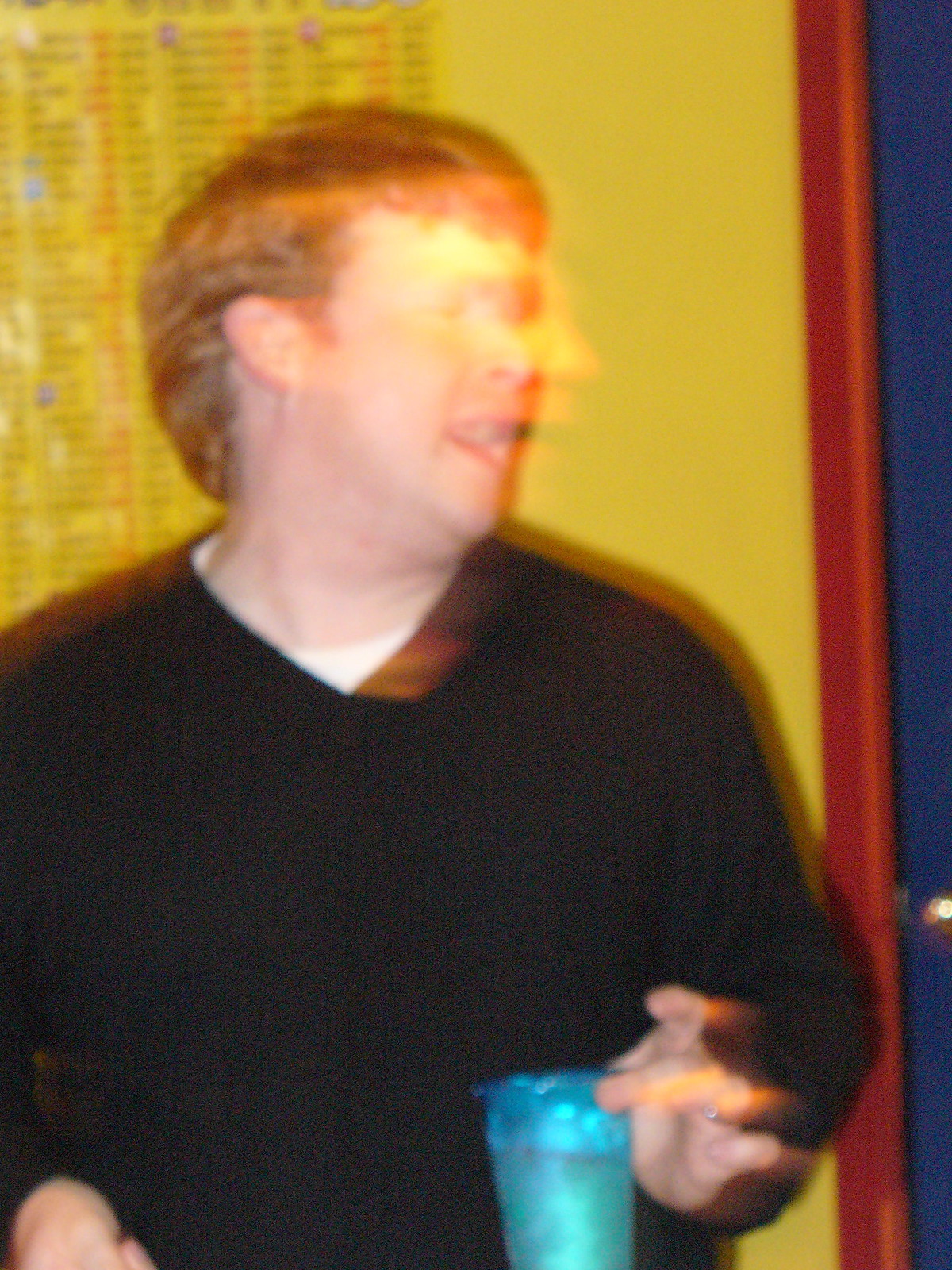The photograph is extremely blurry, depicting a Caucasian man with short, shiny red hair. He appears to be a young to middle-aged gentleman, possibly in his 30s. He is wearing a long-sleeved black shirt with a small V-neck, revealing a white undershirt underneath. His body faces the camera while his head is turned to the right, captured mid-word, giving the impression of motion blur and a double image effect. In his left hand, he holds a translucent blue plastic cup containing a beverage with ice, gripping it delicately with his middle finger and thumb. Behind him, there is a yellow wall featuring what seems to be small text or a menu, along with a brown wooden door frame to the right and a possibly navy blue section of the wall to the left. The lights around his eyes and nose add a notable detail to the otherwise hard-to-decipher image.